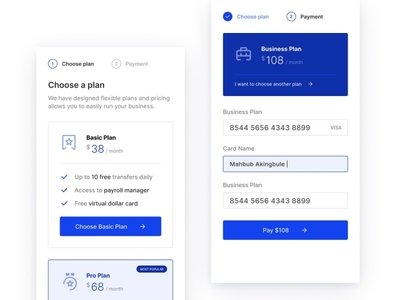The image features a light gray background with two prominent white rectangular sections. 

In the top section, titled "Choose Plan," the design showcases a selection of flexible plans and pricing options to help kick-start a business:

1. **Basic Plan**: $38 per month, accompanied by a list of three features, each marked with a check.
2. A blue rectangle button labeled "Choose Basic Plan" with a right-pointing arrow.

Additionally, there is the **Pro Plan** priced at $68 per month, with a blue circle that contains a check mark next to it and the label "Choose Plan."

In the lower section, distinguished by a circle with the number 2, the text reads "Payment." Below it is a blue rectangle displaying the **Business Plan** priced at $108 per month. This portion further includes fields for entering card details, indicative of the text "Visa" and "card name."

Towards the bottom, another blue rectangle prompts "Pay $108" with a right-pointing arrow.